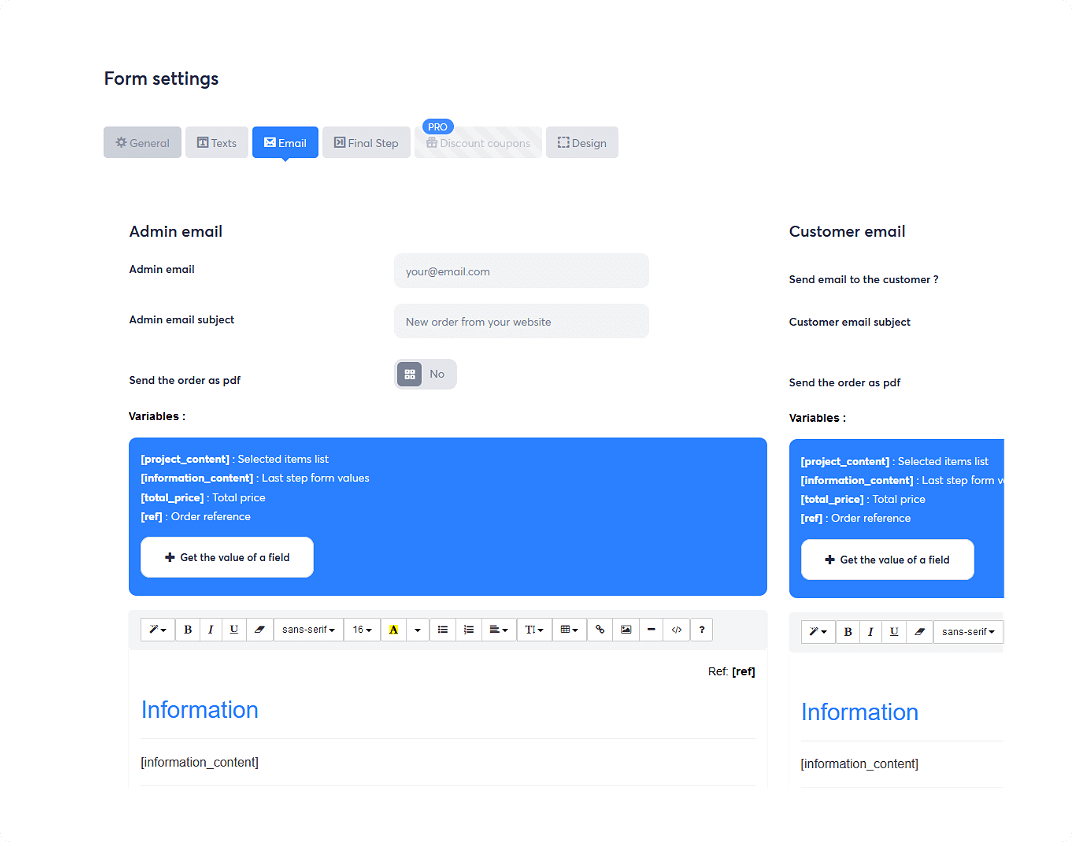Here's a detailed and cleaned-up caption for the described web page image:

---

The image showcases a web page interface focused on email settings. At the very top left corner, there is a label "Form Settings." Below this, six different tabs are displayed horizontally. The third tab, highlighted in blue, is labeled "Email." The other tabs include "General," "Text," "Final Step," "Discount," a hard-to-read label due to faint text, and "Design."

On the left side of the interface, the section starts with "Admin Email," followed by a smaller sub-label "Admin Email" and a text box for input. Below it, there is a label "Admin Email Subject" with an adjacent text box pre-filled with "New order from your website." Further down, there is a toggle option titled "Send the order as PDF" with "Yes" selected. The next section is labeled "Variables," under which a long blue rectangle spans roughly 75% of the way across the width. This rectangle contains small white text listing "Project Content Selected, Items List, Information Content, Last Step from Form Values, Total Price," followed by "Total Price" again. The section concludes with the label "Ref" and "Order Reference." A gray rectangular button below these labels reads "Get the Value of a Field."

On the right-hand side, starting from the top right corner, there is a label "Customer Email" followed by "Send email to the customer?" and "Customer Email Subject." Below this is "Send the order as PDF" and "Variables." Another blue rectangle is present but partially cut off. The visible text within this rectangle repeats "Project Content Selected from List, Information Content, Last Step from Form Values, Total Price, Total Price, Reference, Order Reference." There is another gray button here labeled "Get the Value of a Field."

At the very bottom of the page, running from left to right, is a menu bar similar to what is found in word processing software, offering options like "Bold," "Italic," "Underline," "Font Color," and "Paragraph." Beneath this menu on the left side, "Information" is highlighted in blue with "Information Content" in black underneath. The lower right corner mirrors this with "Information" in blue and "Information Content" in black.